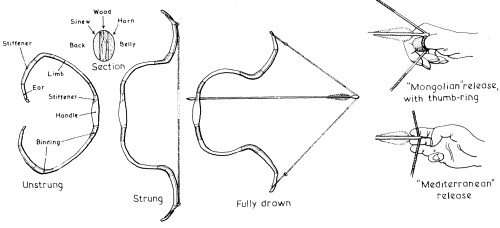The hand-drawn black and white diagram provides a detailed demonstration of different bow usage techniques and bow components. On the left side, there are three distinct diagrams of a bow, starting with a depiction labeled "unstrung" that resembles a backward C. Key parts such as the ear, stiffenings, limb, stiffener, handle, and binding are labeled in a clockwise manner. The middle diagram shows the bow in a "strung" state with curved edges, and the rightmost diagram illustrates the bow "fully drawn" with an extended string and an arrow ready to be shot. The detailed breakdown of the bow includes materials like wood, sinew, and horn, as well as specific parts like the limb and handle.

On the right side of the image, there are two smaller diagrams focusing on hand positioning for drawing the bow. The top diagram shows the "Mongolian release with thumb ring," while the bottom diagram demonstrates the "Mediterranean release." Both diagrams highlight the hands pulling back the string, providing a clear visual guide on how to properly hold and release a bow using different techniques.